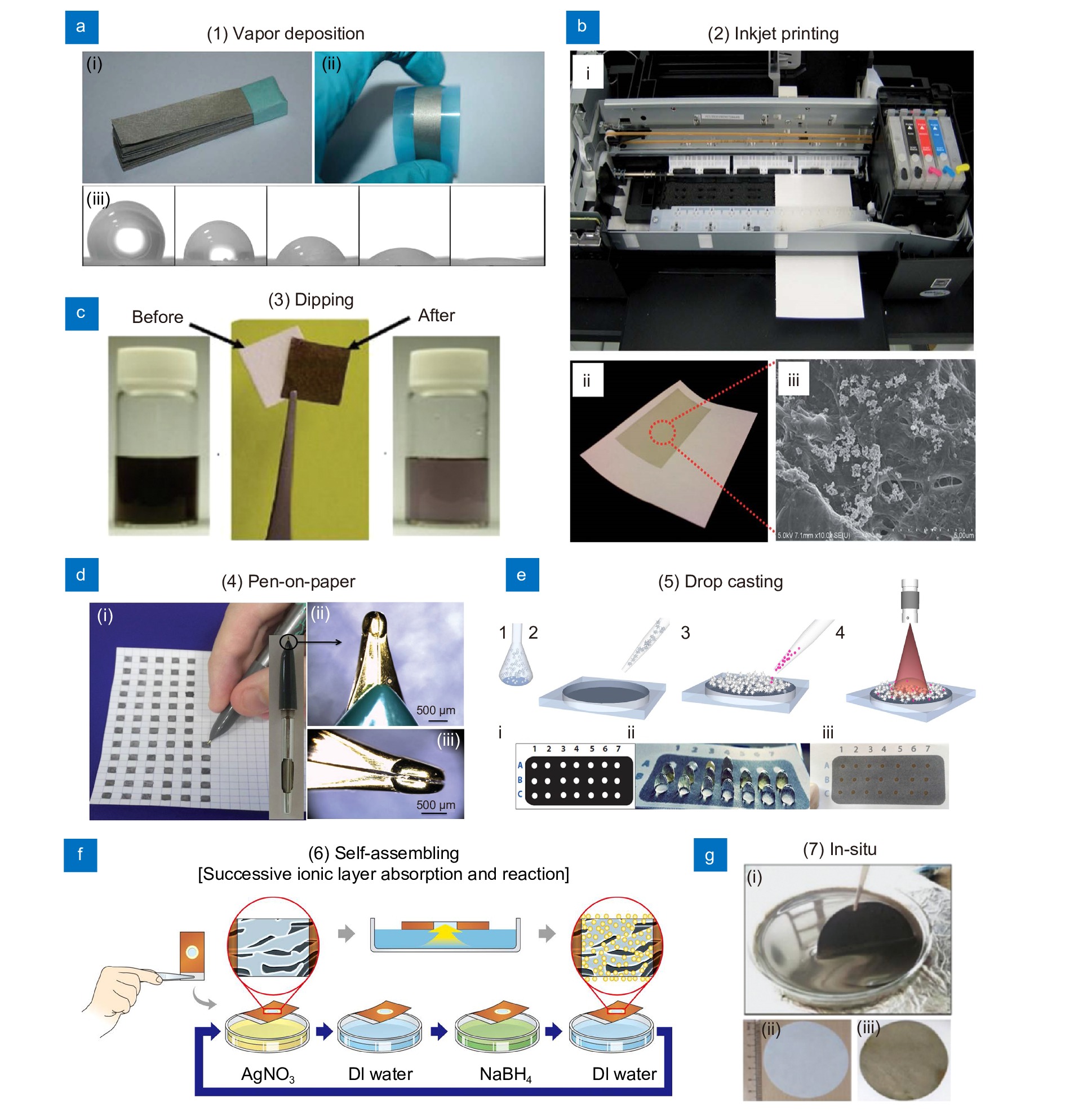The image is a detailed infographic combining text, photographs, and illustrations, segmented into sections labeled from A to G. These sections represent different scientific and technological processes:

- **A: Vapor Deposition** – This section features a series of three parts, illustrating the steps involved in vapor deposition. It shows a stack of papers possibly held together by blue paper, a gloved hand bending a strip of paper, and a sequence of five boxes demonstrating a flattening bubble shape.
  
- **B: Inkjet Printing** – This shows the inner workings of an inkjet printer. Accompanying images include one of the printer itself, a close-up of a piece of paper with a highlighted section, and a grayscale close-up of the printing process.

- **C: Dipping** – Depicts a "before and after" scenario. The images include a material both pre- and post-dipping process.

- **D: Pen on Paper** – Features a gray pen, possibly a fountain pen, writing on graph paper with close-ups of the squares being filled in.

- **E: Drop Casting** – Illustrated through showing a beaker, a dropper, and sequences of droplets being added to and tested on paper strips labeled with a grid (rows labeled A-C and columns 1-7), demonstrating the controlled process of drop casting.

- **F: Self-Assembling (Successive Ionic Layer Absorption and Reaction)** – Presented with illustrations showing a hand using an eyedropper to add solutions like AGNO3, DI water, and NABH4 into Petri dishes. The Petri dishes exhibit various stages, with detailed blow-ups of specific changes.

- **G: In Situ** – Depicts a bowl containing a liquid that appears metallic. Additional images include a Petri dish setup involving paper circles at different stages, highlighting changes in appearance from gray to dark brown.

This collective series of images and descriptions highlights various intricate scientific processes, each visually documented with respective tools, materials, and results in a detailed and educational manner.